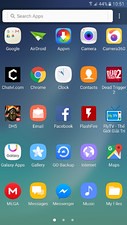The image showcases the home screen of a smartphone with a striking blue and green ombre background. The phone itself is not visible beyond the screen's display. At the top of the screen, a search bar is present, and to the right, icons indicate battery life, Wi-Fi connection, and the time, though it's not discernible from the image. 

The home screen is organized into five rows of app icons in various colors. Among these, the Facebook app is prominently located towards the middle, easily recognizable by its blue square with a white "f." The Google app is also visible, sporting its iconic multi-colored "G" logo in yellow, green, blue, and red. 

At the bottom of the screen, a red circle with a white "M" signifies the presence of the Gmail app. Additionally, a music app featuring a musical note icon and a Maps app, likely the Apple Maps app, are present. 

Other notable apps include one with a red box and a lightning bolt and another with a blue icon featuring a white star in the center. Numerous other apps fill the screen, contributing to a visually diverse and well-organized home screen.